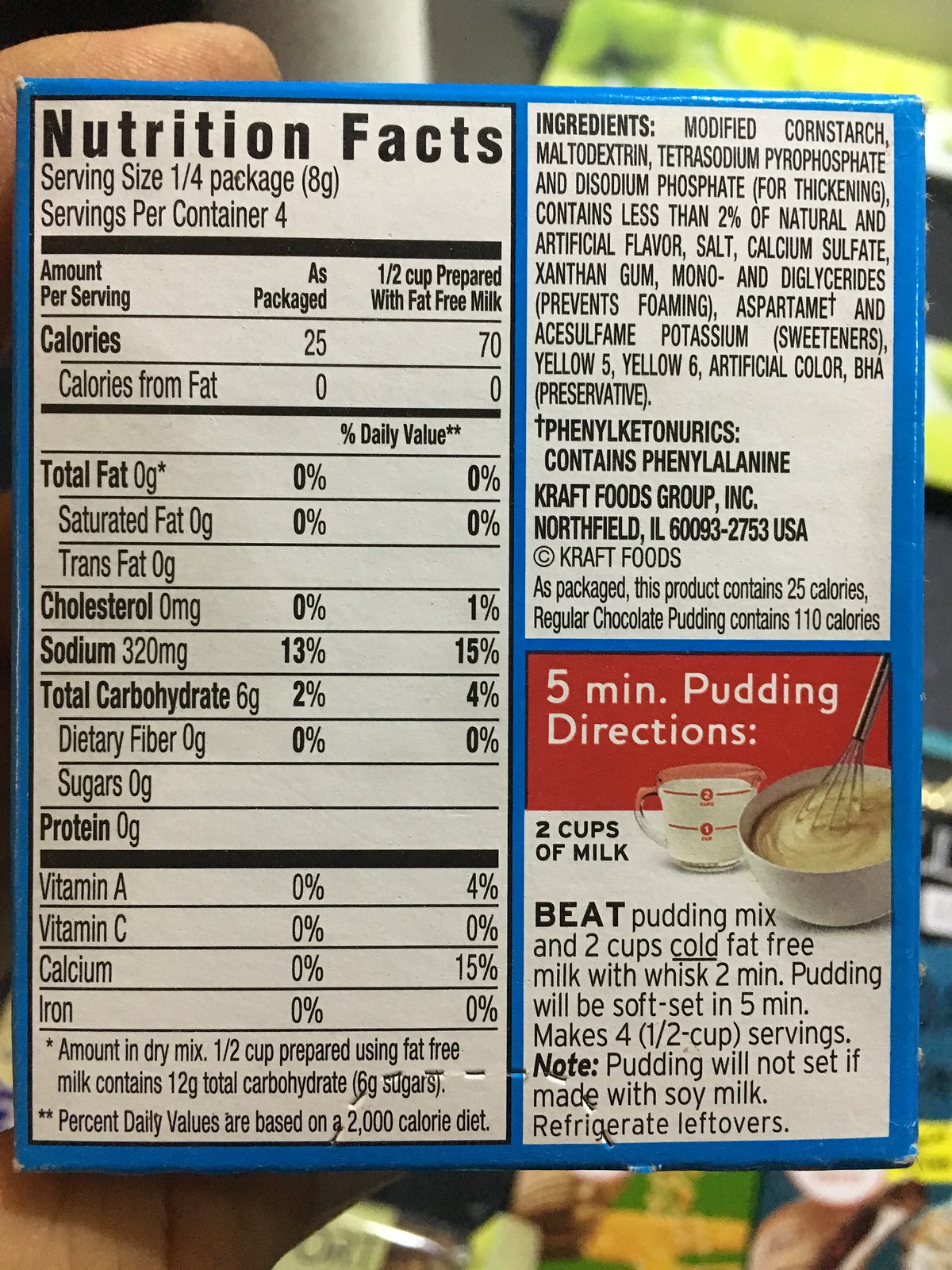The image is a close-up view of the back of a blue pudding package produced by Kraft Foods Group Incorporated, located in Northfield, Illinois, USA. Prominently displayed is a black nutritional facts panel that provides detailed information about the pudding's nutritional content. The panel includes specifics on the serving size, number of servings per container, calorie count, total fat, cholesterol level, sodium, total carbohydrates, protein content, and various vitamins. Below the nutritional facts, there is a comprehensive list of ingredients. In the bottom right corner, a red and white panel offers a quick and easy 5-minute pudding recipe. The packaging features a convenient pull-open tab along a perforated edge on the lower part, designed for easy access.